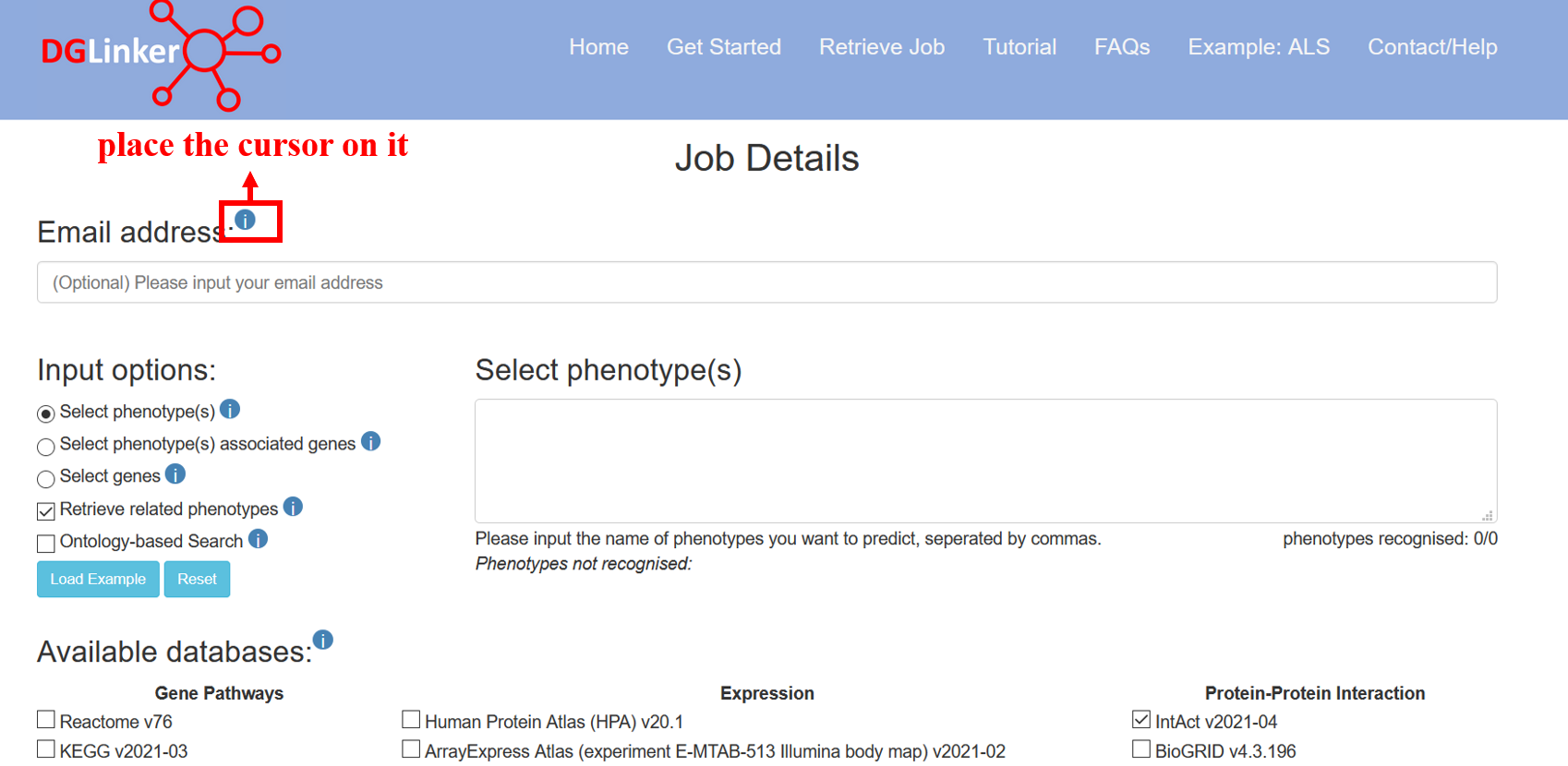The image depicts a webpage featuring a user interface for a bioinformatics tool. At the top of the page, there is a blue banner on the left and red on the right. The banner displays the text "DG linker" in white, with a red logo spread across the top of this banner. Below the banner, there are navigation buttons in white for Home, Get Started, Retrieve Job, Tutorial, FAQs, Example, ALS, Contact, and Help.

Beneath the navigation bar, on a white background, the heading "Job Details" is centered at the top. On the left of this section, there is a field labeled "Email Address" with a button that has a red box around it and an arrow pointing up. The text above this arrow in red reads "Place cursor on it." Below this are the labels: Input Options, Selected Phenotypes, Selected Phenotypes Associated Genes, Selected Genes, Retrieve Related Phenotypes, Ontology Based Search, and Available Databases.

The main body of the image features a large, empty text box where users can input data. Above this box, the instruction reads, "Selected phenotypes." Below, it prompts users to "Please input the name of phenotypes you want to predict, separated by commas." Additional information shows "Phenotypes not recognized" and "Phenotypes recognized: 0/0." Toward the bottom, there are references to data sources such as "Expression: Human Protein Atlas, Array Express Atlas in ACT v 2021-04" with "Biogrid v4.3.196" being the selected database.